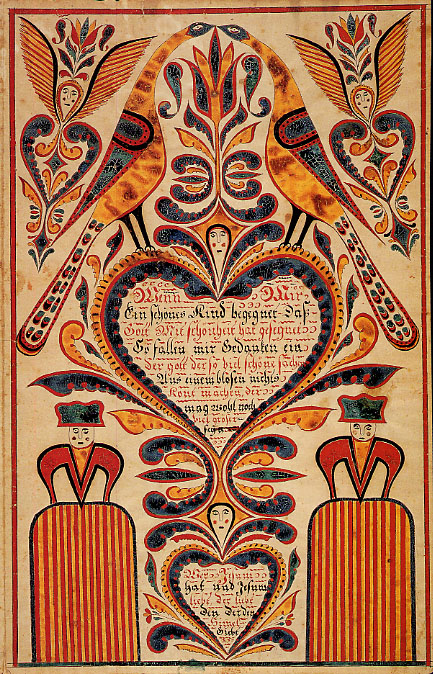The image is a detailed, vibrant tapestry featuring a vertical, rectangular format with a light beige or cream background. It is bordered by red on three sides and black on the bottom. Dominating the top half are two golden-brown birds with blue heads, depicted in profile and touching beaks, standing on a central heart-shaped design filled with old-timey red and black script in an unreadable foreign language. The primary colors throughout the tapestry are gold, red, light blue, and dark blue, adding rich detail and depth.

Encircling the heart and the birds are intricate designs and patterns. Notably, there are six pairs of humanoid faces adorned with hat-like feather decorations, resembling jacks from a deck of cards. These faces are integrated into heart-shaped motifs that mirror each other from left to right. There are also additional heart and floral designs interspersed throughout the tapestry.

At the lower section of the tapestry, there are two small figures—positioned on the right and left—holding a striped red and yellow sheet, which may resemble podiums. These figures have detailed upper bodies and wear distinctive hats, contributing to the intricate and symmetrical aesthetic of the artwork.